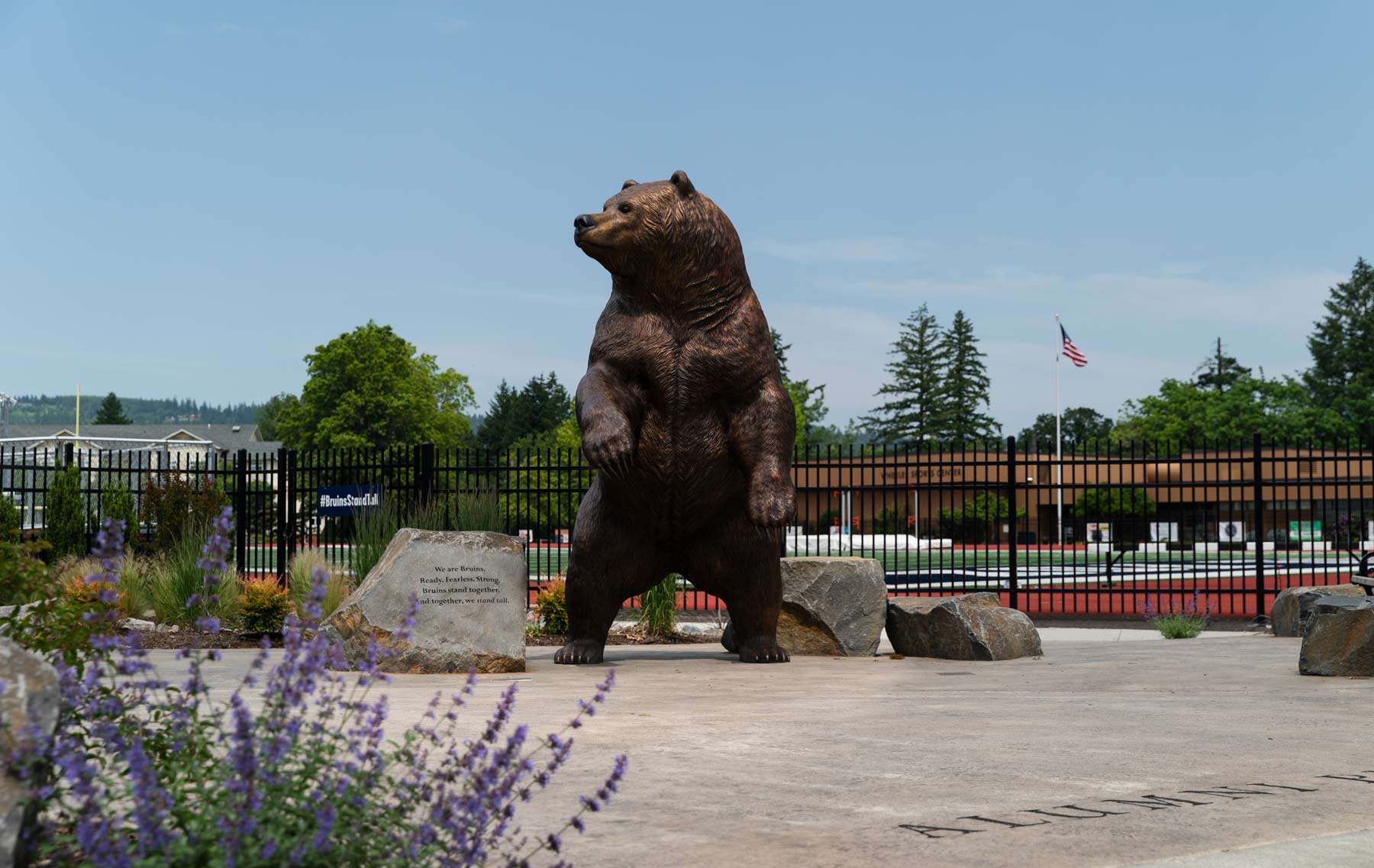This photograph, taken on a sunny day in the United States, features a large bronze statue of a bear standing on its hind legs. The bear, which appears to be between 12 to 15 feet tall, is attentively looking to its right, with both paws raised as if in an attack stance. At the base of the statue is a concrete foundation where a prominently featured lavender bush blooms in the lower left-hand corner of the image, out of focus to emphasize the statue. Next to the bear, two stones bear inscriptions; one reads "We are Bruins, ready, fearless, strong. Bruins stand together, and together we will fall." Behind the statue is a simple black metal fence, behind which an American flag is visible along with various green trees and several buildings, including one with a distinct brown flat roof. A blue sky with light clouds fills the upper half of the image, casting a bright, welcoming light on the scene, which appears to be part of a college campus, hinted by the inscription and the #BruinsStandTall sign on the fence. The word "alumni" can also be seen at the very foreground of the image, reinforcing the academic setting.